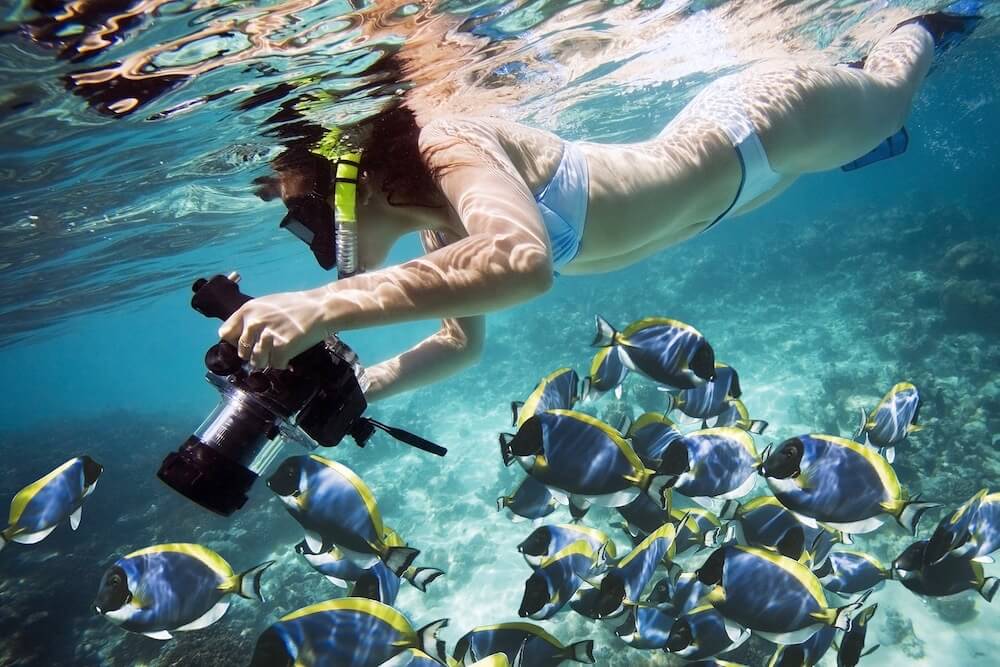An underwater photograph showcases a woman snorkeling mid-swim in crystal-clear, vivid blue water. She is wearing a light blue bikini, accented by dark blue fins on her feet, and is equipped with a black snorkel mask featuring neon yellow tubing extending above the water surface. The woman is holding a large underwater camera encased in a combination of black and see-through plastic, which she grips with both hands.

Beneath her, a school of roughly twenty vibrant fish swims in unison. These fish have striking blue bodies, black faces, bright yellow dorsal fins, and fins with black and white markings. The underwater scene is bathed in a bluish hue, enhanced by the sun's rays filtering through the rippling surface, illuminating the colorful aquatic life below. The water reveals a delicate blend of teal and light blue shades, with hints of gray-green rocks scattered on the bottom, creating a serene and picturesque underwater landscape.